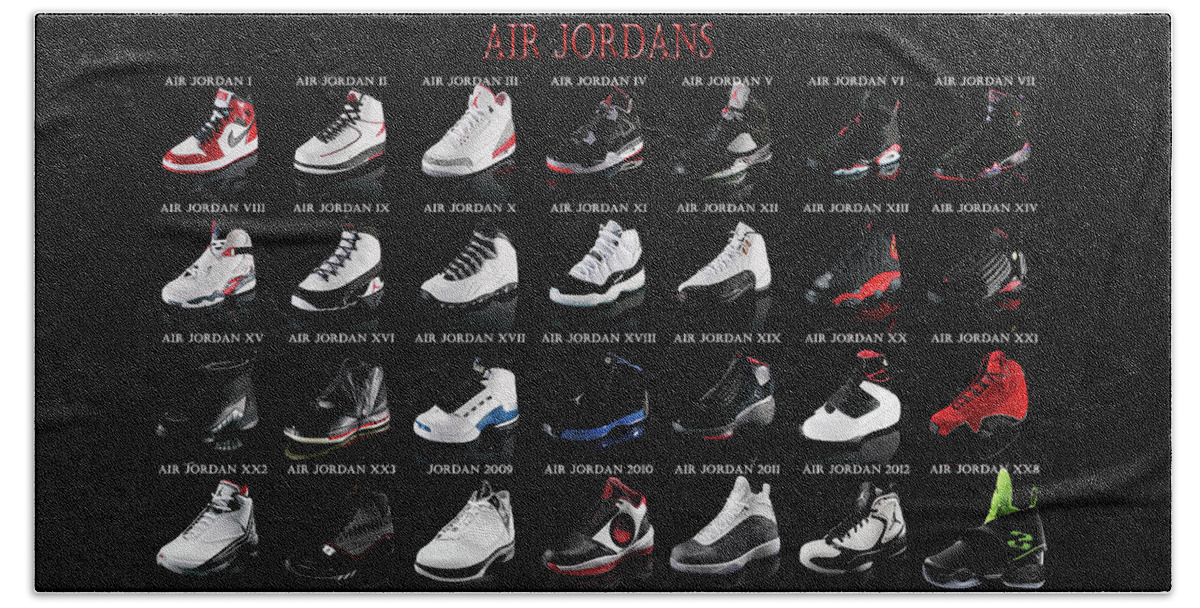This photograph features a cloth banner titled "Air Jordans" in bold red capital letters. The banner showcases a comprehensive history of Air Jordan shoes, arranged in a grid format with four rows and seven columns, totaling 28 different models. Each row starts with the earliest models, beginning with the Air Jordan 1 at the top left, and continues sequentially to the Air Jordan XX8 situated at the bottom right. The shoes are displayed against a black, leather-textured background. The Air Jordan 1 is prominently white and red with black laces and the iconic Nike logo, while the Air Jordan XX8 stands out with its significantly taller profile, predominantly black color, and minimal green accents. The visual comparison highlights the evolution in design and aesthetics of the Air Jordan lineup over the years.